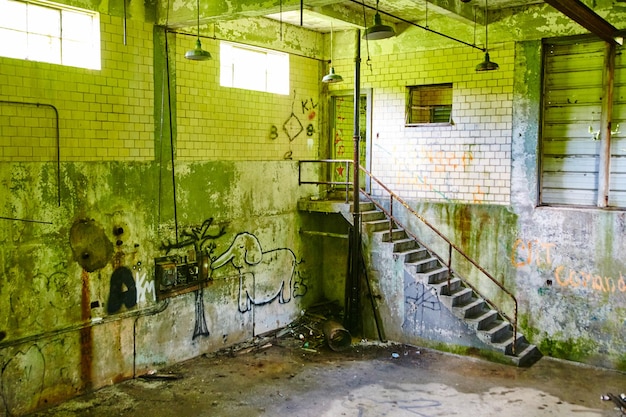The image depicts a grungy, abandoned mechanic's area or an old repair shop located in the basement of a building. The overall environment is very dilapidated and neglected, characterized by shades of gray, brown, and a yellowish-green hue. The concrete floors are littered with trash, particularly in the corners, and show signs of dampness and dirt. The walls, constructed of both white breezeblock and concrete, display significant wear and decay. Distressed areas feature rust stains, brown spots, and patches of moss or mildew. Graffiti is prevalent throughout, with notable artwork including an elephant and various writings across both lower and upper levels. The area showcases two high windows on the left wall, with a small doorway flanked by concrete steps. There is a high, square hatch between the door and what seems to be a loading bay, suggesting it might have been a delivery area. Industrial features include three high-hanging lamps with dark green shades suspended from the ceiling. The overall scene is desolate and unwelcoming, marked by broken-down elements and an overall sense of abandonment.